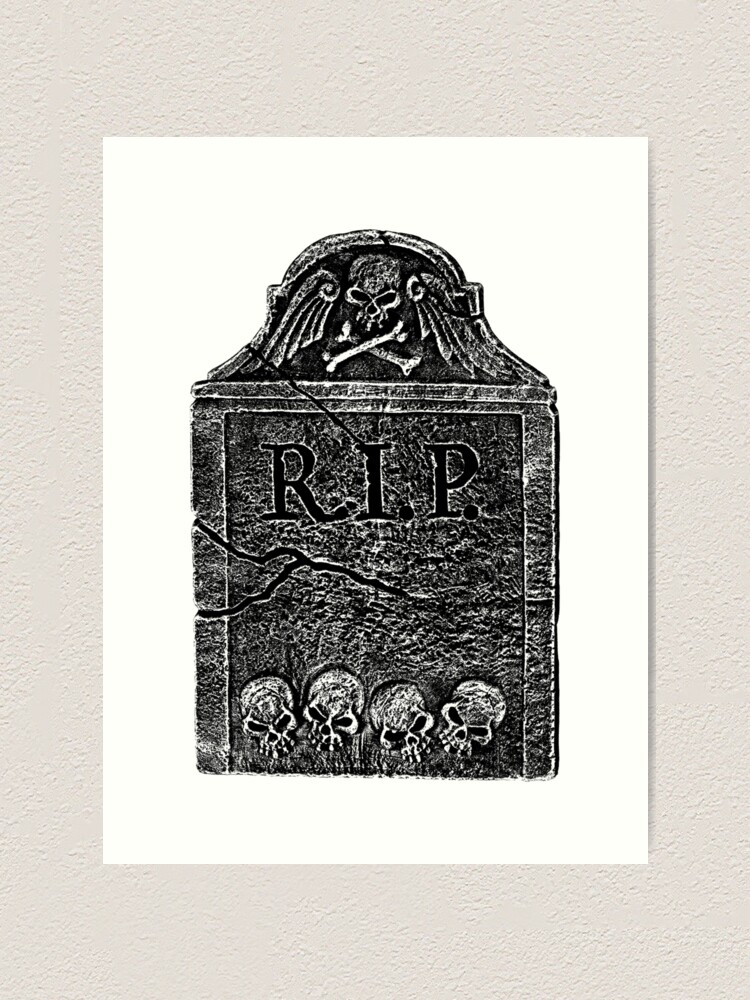This image shows a white piece of paper with a black and gray ink print of a gravestone, mounted against a textured, beige-colored background. The gravestone features a central motif of a skull with wings extending from either side and crossed bones beneath it. The top of the gravestone prominently displays the letters "RIP" in all capitals. The tombstone also bears visible cracks, both in the middle and near the top, adding to its weathered and eerie appearance. At the bottom of the gravestone, there are four smaller skulls arranged in a row. The entire composition, highlighting elements such as the dark skulls and the intricate cracks, conveys a slightly creepy and somber atmosphere.